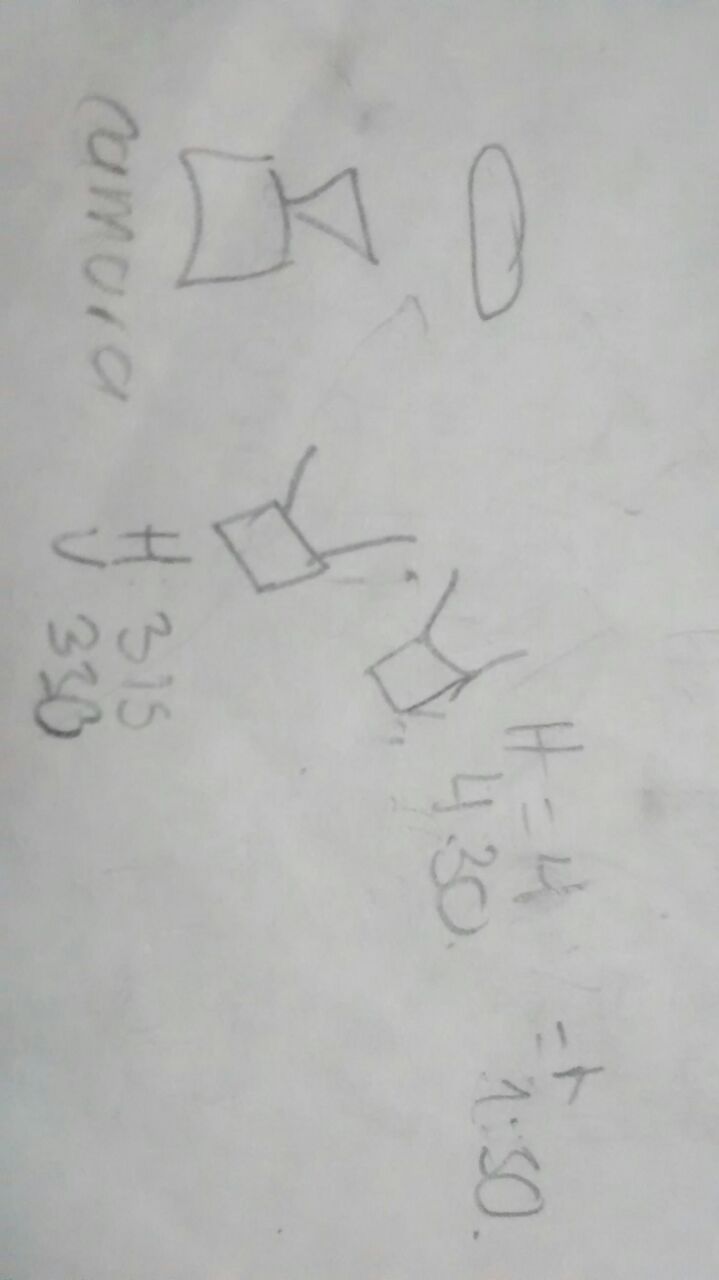In this photograph, we see a white sheet of paper featuring handwriting in a light gray tone, likely made with a pencil or a softly colored pen, as it is not dark enough for black ink. The writing appears to be oriented sideways, requiring the viewer to tilt their head to read it correctly.

At the top of the image, there is a circle, followed by a gap, then a triangle adjacent to a square. Next to these shapes, the word "Camaro" is written, spelled out as C-A-M-A-R-O. Below these figures, there is a square with two curved lines extending from its top, resembling antennas. To the right, after a couple of inches of space, there is another identical square with similar antenna-like lines.

Further down, the letters "H" and "U" are present, each associated with numbers: "H" is paired with the number 315, while "U" corresponds to 330. At the bottom of the sheet, there is a mathematical expression reading "H = 4430 = R130," with the digits similarly aligned sideways.

Overall, the arrangement and the variety of symbols and numbers suggest a visual puzzle or a complex diagram, inviting an analytical interpretation.